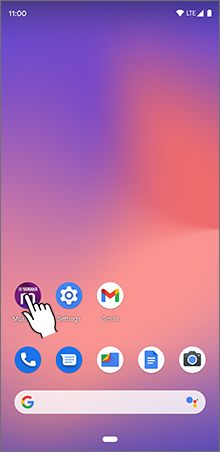The image captured from a cell phone showcases a vibrant interface with intricate details. The background features a gradient of purple with touches of pink towards the middle and bottom. In the top left corner, the time is displayed as "11 o'clock". The top right corner contains the Wi-Fi symbol, followed by "LTE" in capital letters, a small triangle icon, and a fully charged battery indicator.

On the lower half of the screen, there are three circles aligned in a row. The first circle is purple with white writing inside, depicting a white hand with the index finger pointing at the circle, and the word "Music" underneath. Next is a blue circle containing a white gear icon labeled "Settings". The third circle is white with a multicolored M that represents Gmail.

Below this row, there is another line containing five circles. From left to right: a blue circle with a white telephone icon, another blue circle with a white sheet of paper icon, a white circle with a folder icon, a white circle with a blue piece of paper icon, and finally, a white circle with a camera icon. At the bottom, a blue bubble rectangle with a prominent capital "G" on the left-hand side completes the visual composition.